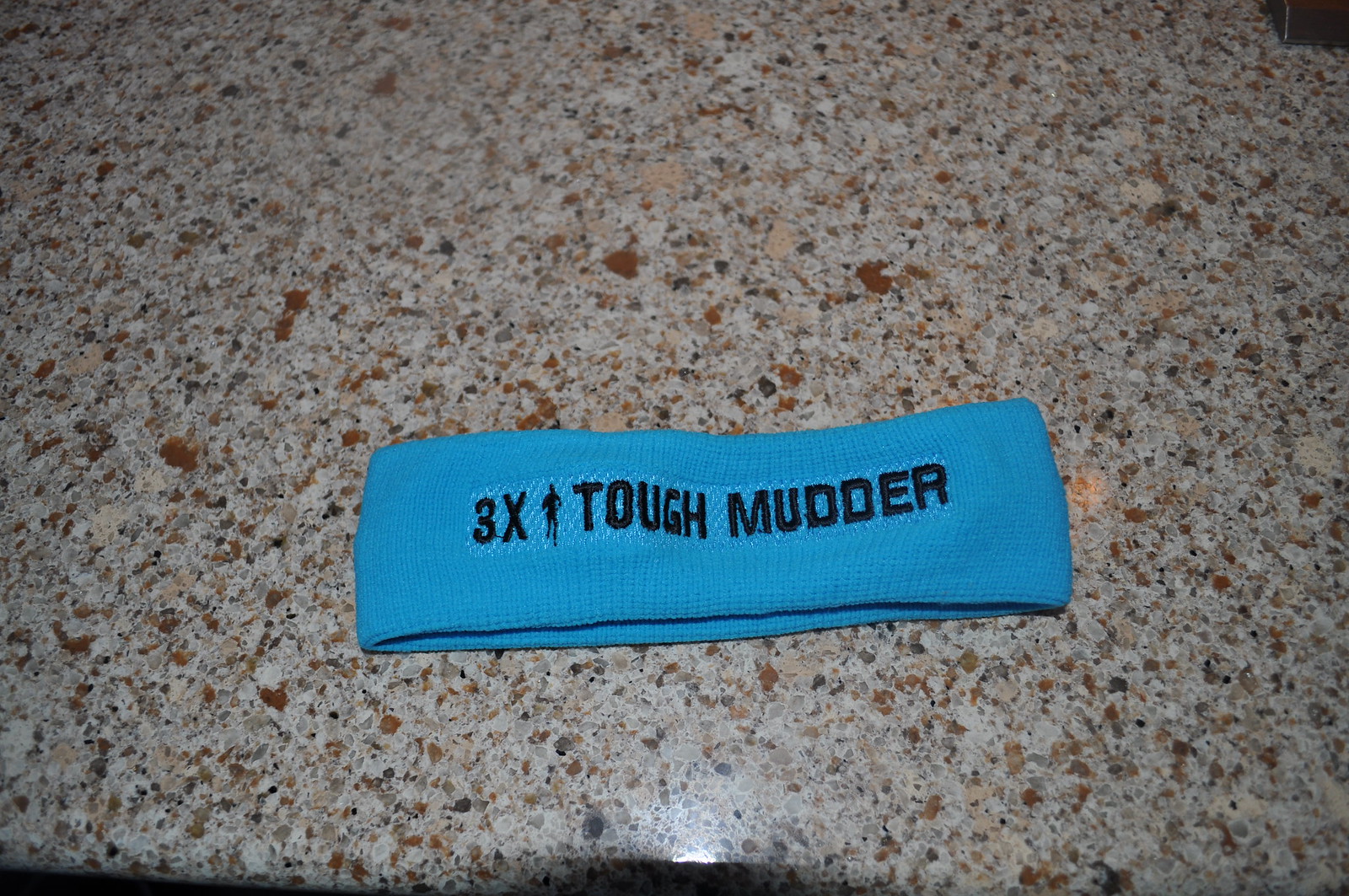This color photograph, taken in landscape mode, showcases a bright blue athletic sweatband folded in half and laid flat on a smooth, shiny, granite-like countertop. The countertop, tan in color with flecks of chocolate brown, darker tan, white, black, and dark blue, creates a sand-like appearance. A small speck of white light reflects off the bottom center of the marble surface. The sweatband, positioned horizontally, features black text that reads "3X" followed by a small silhouette of a person running and "TOUGH MUDDER" in all caps. The band appears elastic and could likely be worn on the wrist, foot, or leg, emphasizing its versatile athletic use.